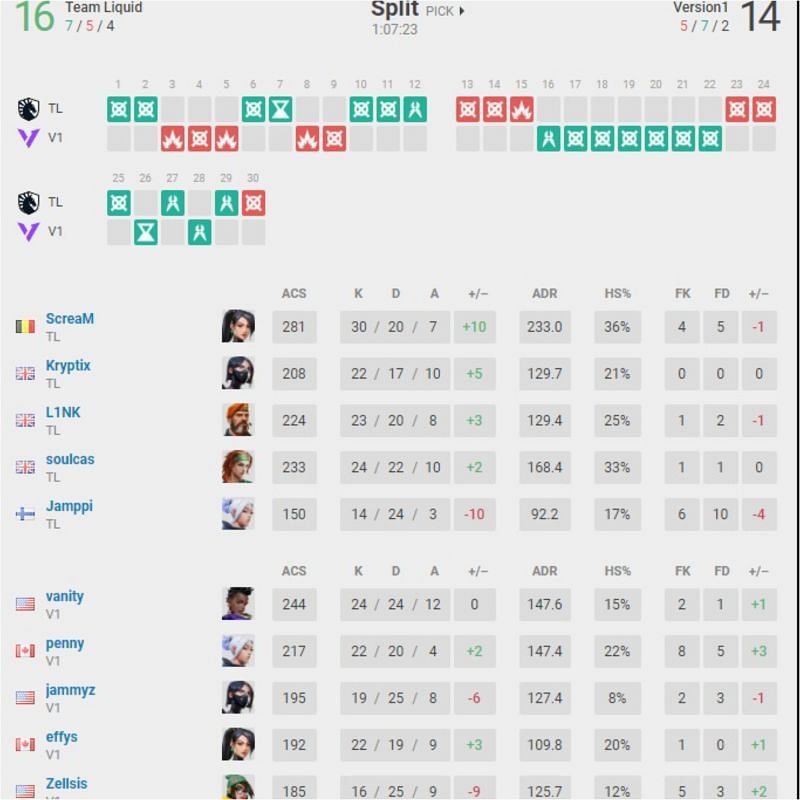This image depicts a detailed scoreboard from an eSports event, featuring intricate statistics and visual elements that outline the performance of different teams and their players. At the top of the page, there are team standings for "Team Liquid" on the far left and "Version 1" on the far right. "Team Liquid" has accumulated 16 points, indicated in green, with a record of 7 wins (green), 5 losses (red), and 4 ties (black). "Version 1" has 14 points, noted in black, and a record of 5 wins (red), 7 losses (green), and 2 ties (black).

The top section of the page is divided into two lines with date ranges; the first line covers dates from 1 to 24 and the second line from 25 to 30. Next to these dates are various icons and two-letter acronyms. For instance, "Team Liquid" is abbreviated as "TL" and represented with a shield icon featuring a horse. The score outcomes include various abstract symbols such as an 'X' with a circle, an hourglass, pliers, a circle with a crosshair, and a fire symbol, possibly indicating different competitive outcomes or game elements.

Below the main scoreboard is a table organized by team and player names. Each row includes various statistical categories labeled as ACS (Average Combat Score), K (Kills), D (Deaths), A (Assists), +/- (Plus/Minus Ratio), ADR (Average Damage per Round), HS% (Headshot Percentage), FK (First Kills), and FD (First Deaths). The team affiliation is indicated in the first column with abbreviations such as "TL" for Team Liquid and "V1" for Version 1.

Overall, the image is a comprehensive snapshot of an eSports competition, showcasing player and team performance through a variety of detailed statistics and visual indicators.